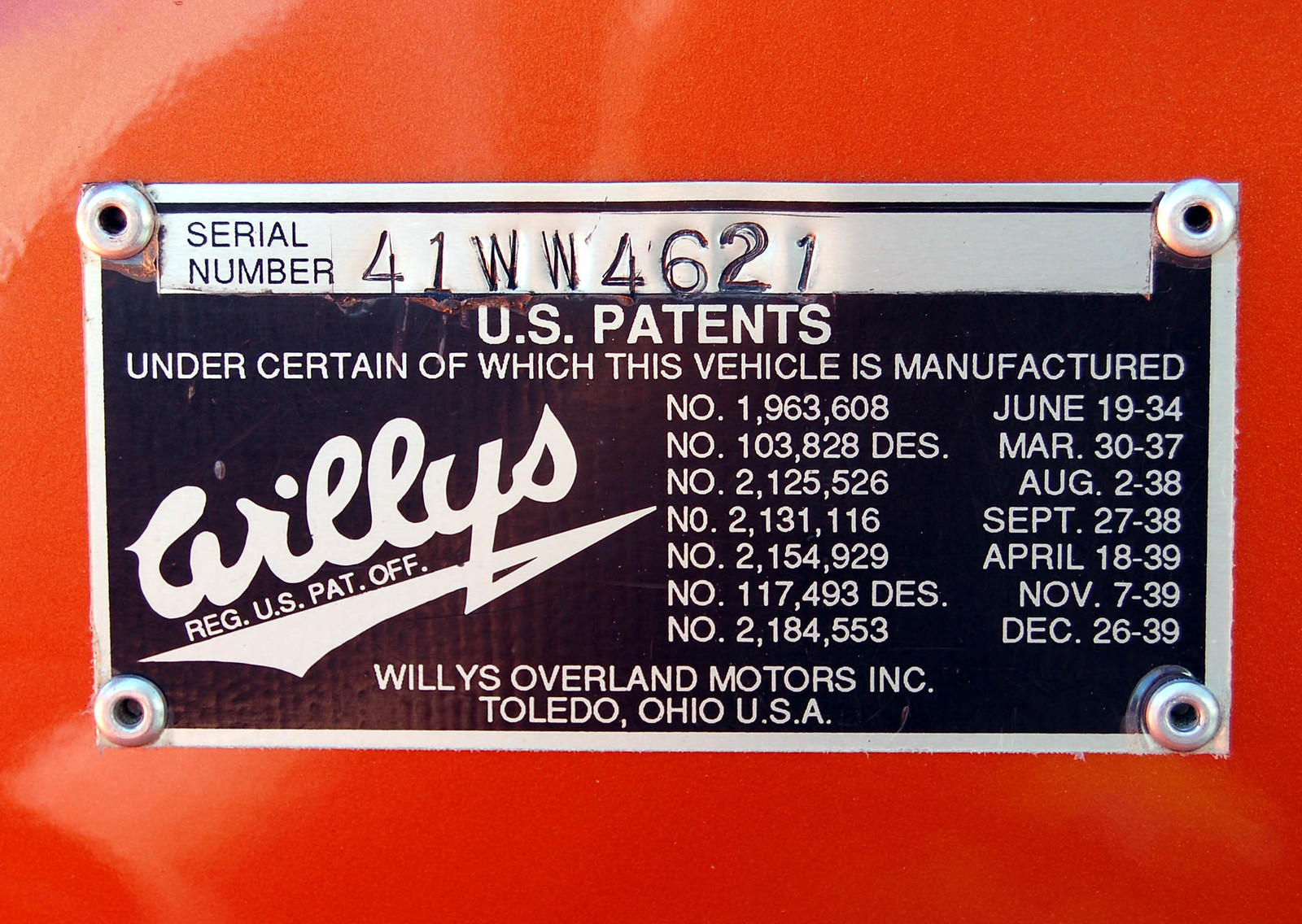This is a detailed, close-up photograph of a horizontal, rectangular black metallic tag affixed to a red surface. The background, entirely red, shows lighter tones in the upper left and bottom left corners due to reflections of white light. The tag is held in place by four silver circular fasteners at its corners. In the unpainted silver section at the top of the tag, the serial number "41WW4621" is inscribed. Below this, in a black painted area, white text reads "US Patents under certain of which this vehicle is manufactured." Adjacent to this text is a list of seven U.S. patent numbers and their corresponding dates, including "NO. 1963608 June 19, 19-34", "103,828 DES March 30-37", and continuing in this format. To the left of these numbers, the word "Willys" is underlined. Beneath the list, at the bottom of the tag, "Willys Overland Motors, Inc., Toledo, Ohio, USA" is prominently displayed, establishing the manufacturer's identity.